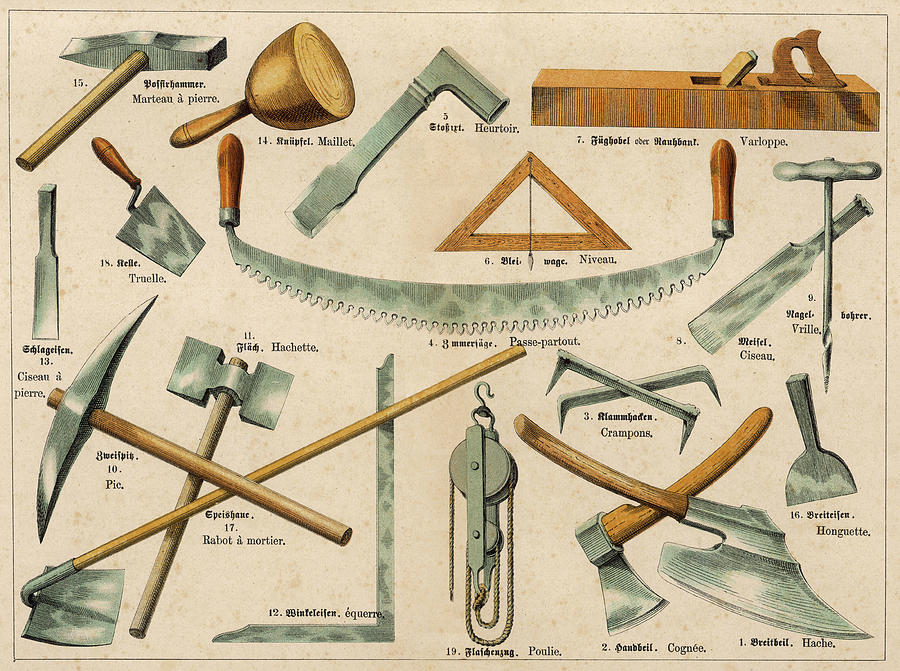A detailed color illustration on weathered brown paper depicts a vintage array of various garage tools from what appears to be the 1950s or 60s. The image is bordered by a slight black line and shows a collection of tools laid out and labeled, primarily in a foreign language, possibly French. Tools such as a mallet, trowel, pickaxe, hatchet, and a two-handled saw are meticulously illustrated. Many of these tools feature wooden handles, adding a rustic, old-fashioned charm, while others are predominantly metal. This diagrammatic poster, reminiscent of what might hang in a craftsman's shed or garage, serves as a key to identifying these diverse implements. The overall aesthetic suggests it is a learning aid, emphasizing the detailed identification and function of each tool, absent of any human or animal depiction.